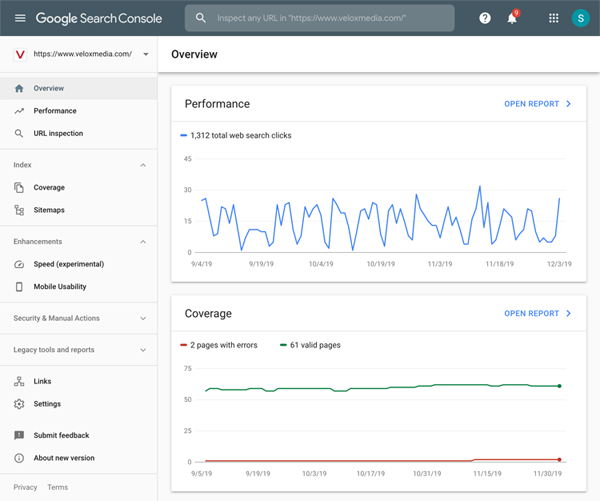The image depicts a screen capture from a digital application, likely Google Search Console. The image frame is slightly horizontally rectangular in shape.

At the top, there is a dark gray horizontal banner with several elements arranged from left to right: 
1. Three horizontally stacked bars for menu options.
2. The text "Google Search Console."
3. A search window.
4. A question mark icon.
5. A notification icon with nine notifications.
6. A square composed of nine white dots.
7. The letter 'S.'

Beneath the banner, on the left-hand side, there is a vertical menu displaying a list of navigational items:
- Performance
- URL Inspection
- Index
- Coverage
- Sitemaps
- Enhancement
- Speed
- Experimental
- Mobile Usability
- Security and Manual Actions
- Legacy Tools and Reports (which includes Links, Settings, and Submit Feedback about the new version)

To the right of the vertical menu, occupying about two-thirds of the frame, is a "Performance" window displaying a blue-lined graph. Below this window, there is another section labeled "Coverage," which features two line graphs, one green and one red.

The detail and arrangement suggest a comprehensive overview of various metrics and tools available within the Google Search Console application, designed for web administrators to monitor and optimize website performance and search visibility.